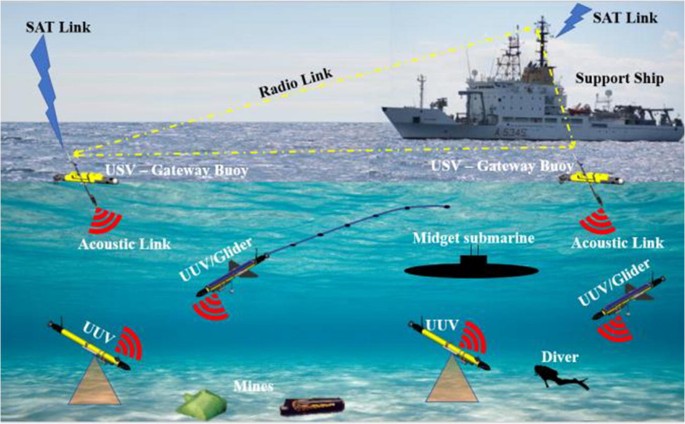The detailed image illustrates a large body of water featuring a ship prominently positioned at the top right, surrounded by a clear, blue, and cloudy sky. The ship is labeled "Support Ship" and "SAT Link," with a blue lightning bolt symbol denoting the SAT Link connection. A line extends from the ship down into the water, marked as "Radio Link," indicating its communication capabilities. Additionally, to the top left of the ship, another SAT Link is indicated with a blue line descending to the water's surface. 

Below the water, the image is meticulously labeled with various subaquatic entities. On the left side, the label "USV-Gateway Buoy" is visible. The ocean floor showcases diverse elements including "Acoustic Link," "UUV/Glider," "Mines," "Midget Submarine," as well as another "UUV/Glider" and "Diver" towards the bottom right. Each of these objects and systems are clearly marked, providing a comprehensive view of both surface and underwater components. The overall artwork is vivid and well-lit, ensuring excellent clarity and detailed representation of the maritime environment.